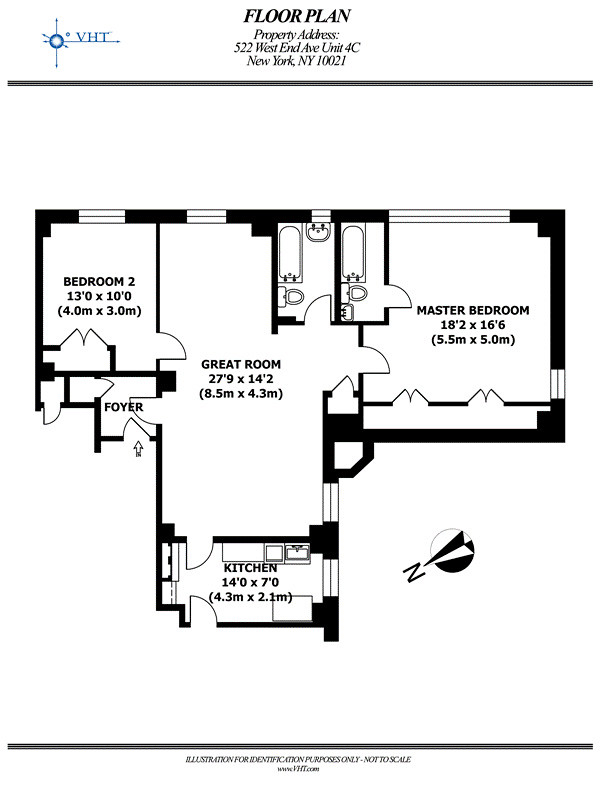A black and white floor plan for an apartment located at 522 West End Avenue, Unit 4C, New York, New York 10021. Positioned prominently at the top center of the image, the address identifies the specific apartment unit. The floor plan details an apartment with a master bedroom, which measures 18 feet 2 inches by 16 feet 6 inches and includes an en-suite bathroom. The layout features a central great room, bordered by the master bedroom and a secondary bedroom, denoted as Bedroom 2. Towards the bottom of the plan, a kitchen is clearly marked. It is important to note that the floor plan is not to scale, as stated at the bottom of the image. Additionally, the illustration is provided strictly for identification purposes only.